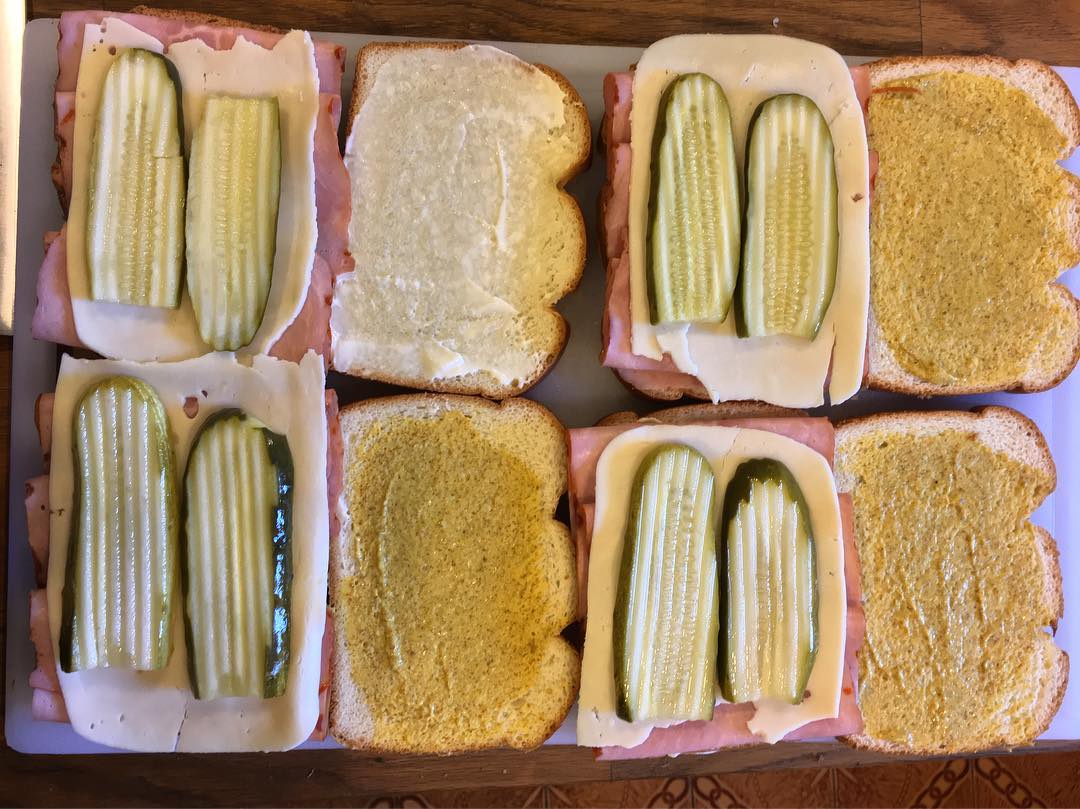This high-definition photograph features eight open-faced sandwiches arranged in two rows on a wooden table covered with what looks like a plastic sheet or wax paper. In each row, there are four slices of bread. The sandwiches are in various stages of assembly, and the ingredients are clearly visible. On each of the sandwiches that include pickles, the long-sliced pickles are layered on top of cheese, which is in turn layered on top of some type of lunch meat, likely ham or turkey.

Starting from the top row, the piece of bread on the top left has ham or turkey, a slice of cheese, and two long slices of pickles. To the right of that, the next piece has a generous spread of mayonnaise. The third piece in this row replicates the first, with meat, cheese, and pickles. The final piece on the top row appears to be spread with mustard.

In the bottom row, the first slice of bread on the left also features meat, cheese, and pickles. The second slice appears to have mustard with visible pepper flecks. The third slice mirrors the meat, cheese, and pickles arrangement. The final piece in this row also seems to be spread with mustard.

The sandwiches are set under good lighting, making all the textures and details, like the spark-like pattern of the mustard and the glossy surface of the pickles, clearly visible. The scene looks like it was taken indoors, possibly during the preparation of a meal. The background reveals the wooden texture of the table and a glimpse of a patterned floor. This well-composed image effectively captures the process of making several sandwiches before they are fully assembled.